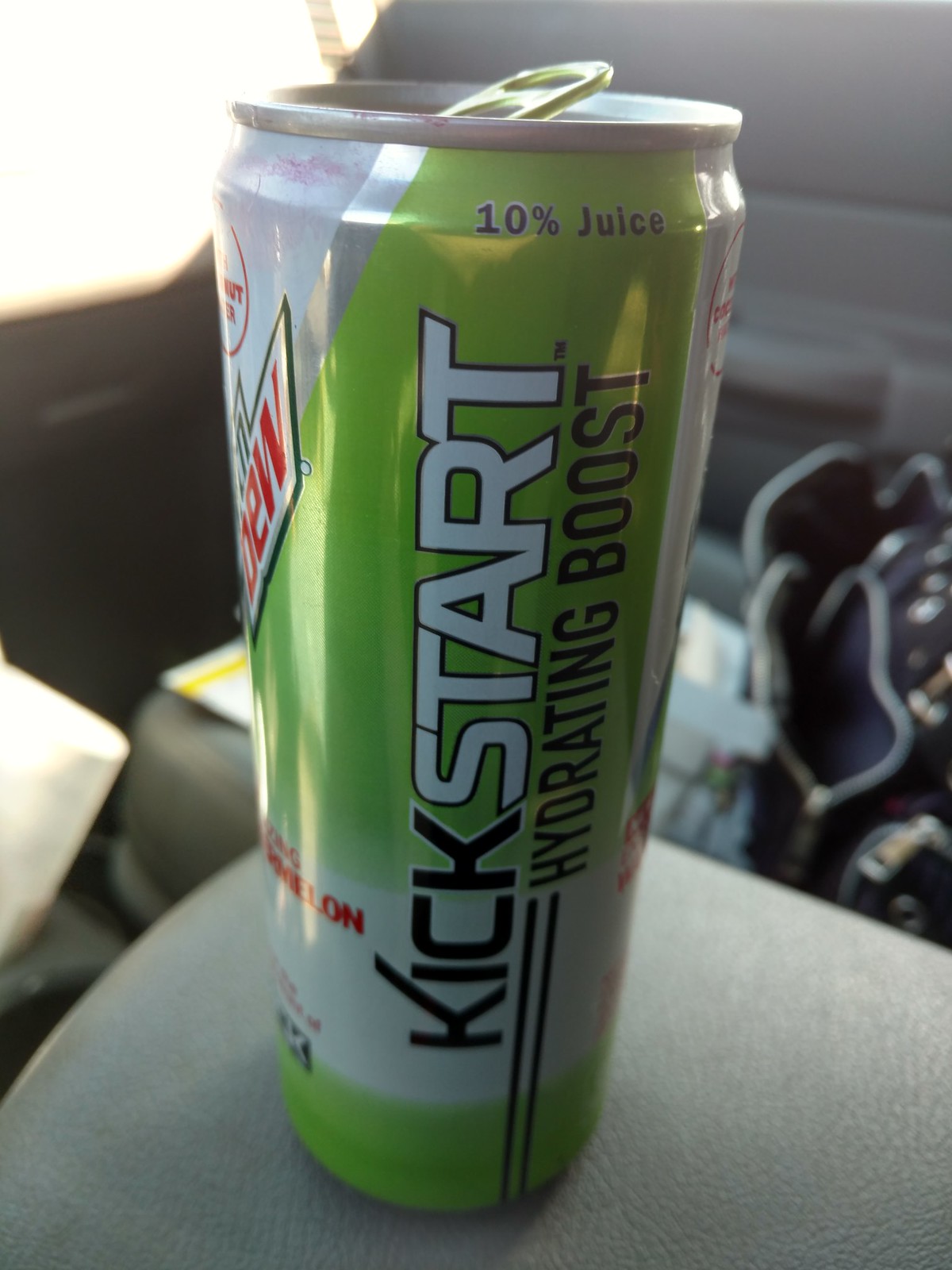In this photograph, a tall metal can of Mountain Dew is prominently featured, positioned on the center console between the two seats of a car. The text on the visible side of the can reads: "Cake Star Hydrating Boost, 10% juice." The can's design includes a light green color with silver accents, and the beverage is identified as some kind of melon flavor. The background reveals a glimpse of miscellaneous items on the passenger seat, adding context to the interior setting. The overall composition perfectly captures an everyday moment within a car environment.